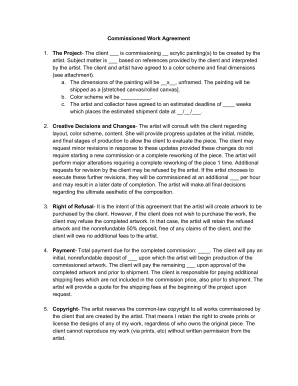The image depicts a "Commissioned Work Agreement" document set against a white background, with black text detailing various categories of the agreement. The categories listed on the document are: 

1. The Project
2. Creative Decisions and Changes
3. Right of Refusal
4. Payment
5. Copyright

Each category is accompanied by a paragraph of text outlining the respective terms and conditions. However, the image is quite small, making it difficult to discern all the details of each section. For example, under "3. Right of Refusal," it is stated that the artist will produce artwork intended for purchase by the client. If the client decides not to buy the artwork, they may refuse the completed piece. Unfortunately, the small print makes it challenging to read the full text clearly.